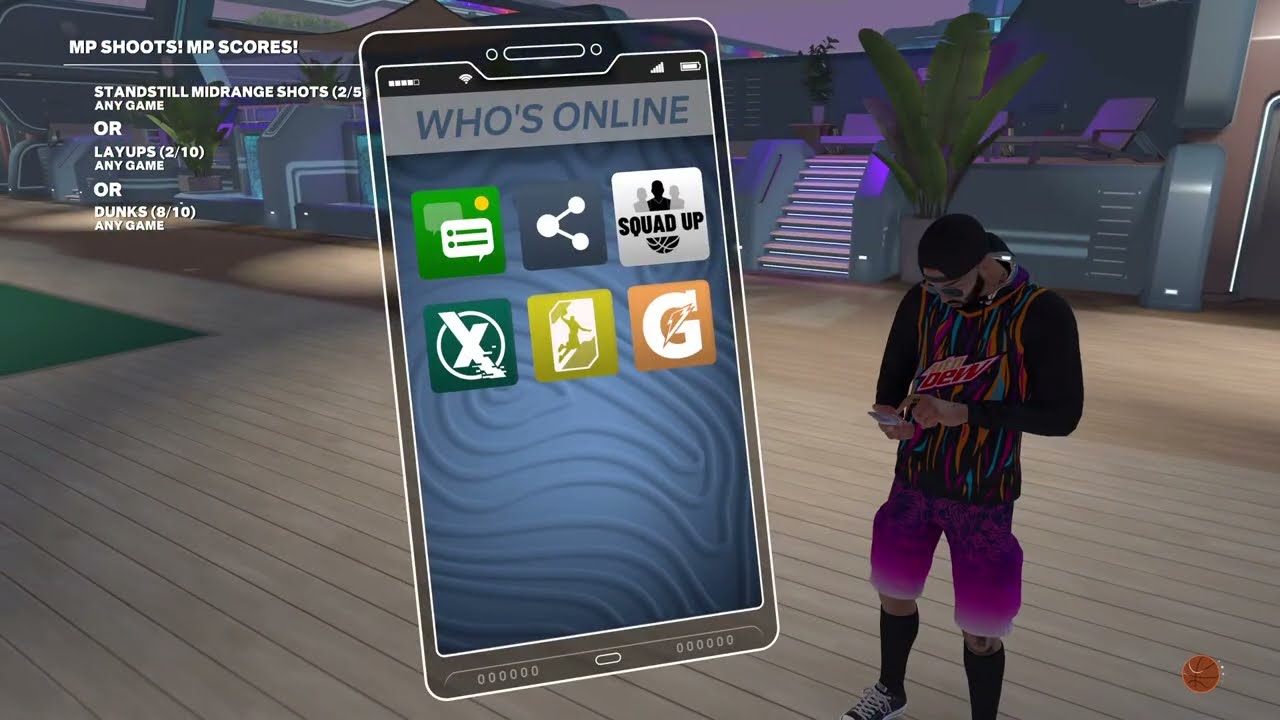This detailed screenshot from a video game appears to depict a scene on what looks like a yacht or boat-like environment with an open area and features such as steps and lights. The top left-hand corner of the screen contains text reading "MP shoots! MP scores!" followed by "stand still mid-range shots any game or layups any game or dunks any game." 

Central to the image is a large depiction of a mobile phone displaying the message "Who's online?" along with several icons including options like "share," an X button, "start a chat," and "squad up." The phone's display is prominently featured on the left side of the screen.

On the right side of the screen stands a character wearing purple pants, a colorful shirt with black sleeves and "Mountain Dew" branding, glasses, and a black cap. This character is looking down at his phone, standing on a wooden plank area with a background that includes consoles, metal boxes, and a potted plant. The scene's sky has a purple hue, suggesting either dawn or dusk.